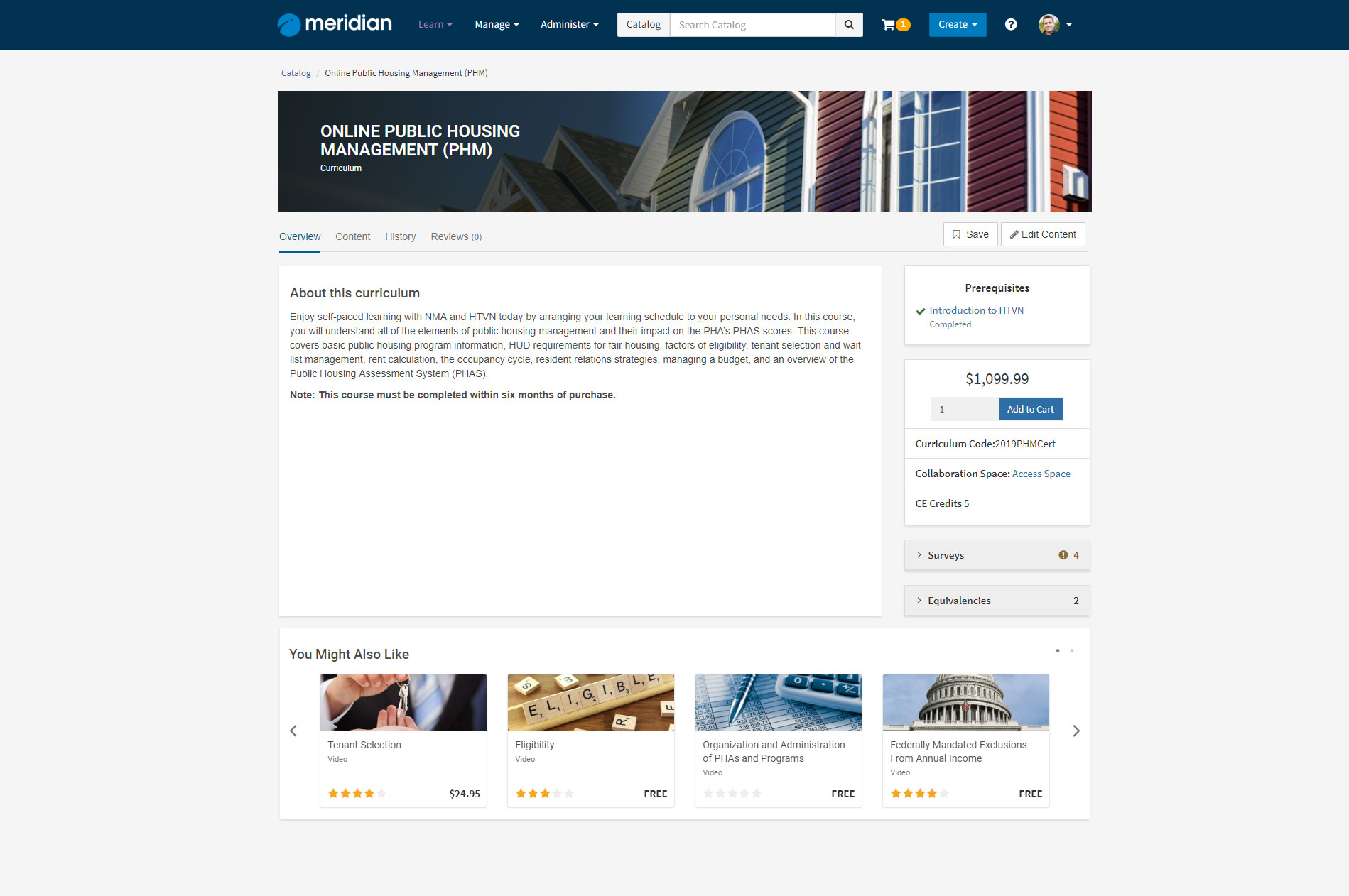Here's a cleaned-up and detailed caption for the image:

---

Screenshot of the Meridian College course page for "Online Public Housing Management." The webpage features several navigation tabs, including "Learn," "Messages," and "Administration," with a search bar and a "Create" tab. The highlighted section details the course, explaining the curriculum and prerequisites. The cost for enrolling in the course is $1,099.99. A small profile picture suggests the course is being viewed by a female student. The page also includes sections for additional resources and recommendations under "You May Also Like."